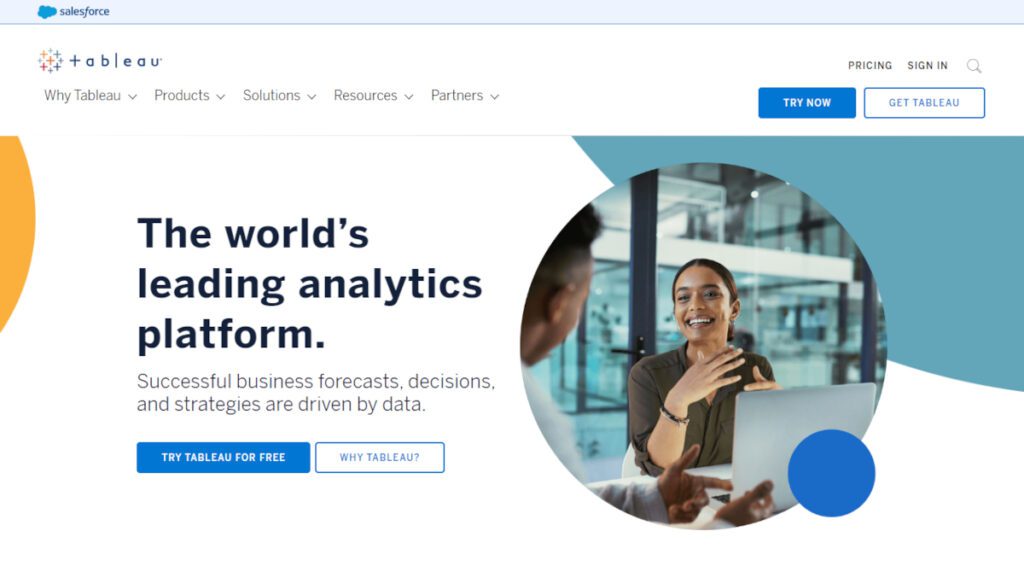The webpage screenshot features a light blue navigation bar at the top, with a cloud-like icon in the upper left corner next to the word "Salesforce," written as a single word. Below this, the rest of the page features a white background. To the left is an icon with multiple plus signs in different colors: dark, red, dark yellow, and orange, symbolizing "Tableau," spelled "t-a-b-l-e-a-u."

On the far right of the top navigation, there are links labeled "Pricing," "Sign In," and a search icon. The following line features several drop-down menus titled "Why Tableau," "Products," "Solutions," "Resources," and "Partners." Toward the far right, there are two buttons: a blue one labeled "Try Now" and a white one with a blue border labeled "Get Tableau."

Below this, the right half of the screen displays an image of a young, light-skinned Black woman with her hair pulled back, wearing a brown shirt. She is smiling and has her hands raised as if she were speaking. In front of her sits a gray laptop. She is conversing with a Black man with short, puffy hair, who is gesturing with his hands.

To the bottom right of this image, there's a round blue circle, and to the left, it reads "The world's leading analytics platform" in dark font. Underneath, the text states, "Successful business forecasts, decisions, and strategies are data-driven." Two tabs follow this: a blue button labeled "Try Tableau for free" and a white one with a blue border labeled "Why Tableau."